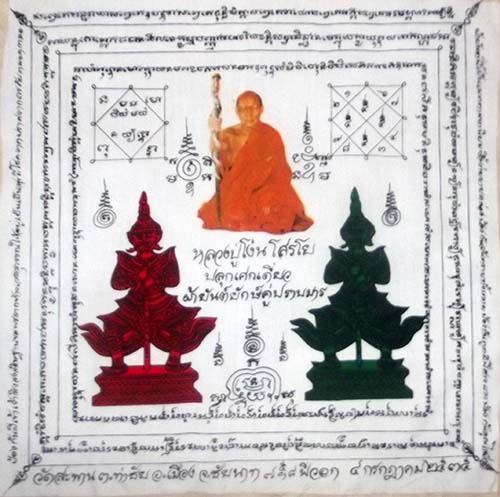The image depicts an ancient, square, illuminated manuscript with a parchment-like background, tinged with brown stains at the edges. The layout consists of three concentric layers of papers with ornate borders and intricate, unreadable foreign text or symbols adorning these layers. 

At the very center, housed within a square border, is a depiction of an elderly, bald, Asian religious figure, likely a Buddhist monk. He is dressed in an orange robe and holds a wooden staff in his right hand, evoking an image reminiscent of the Dalai Lama. The figure appears slightly out of focus, adding to the antiquated feel of the manuscript.

Flanking the central figure are two statues positioned at the bottom left and right corners of the inner square. The statue on the left, perched on a red rectangular base, portrays a man squatting down, wearing a pointed hat and ancient attire, his hands folded in front of him. The statue on the right mirrors this form but is colored in blue-green hues. Both statues resemble soldiers or guardians and add to the spiritual and ceremonial aesthetic of the piece.

In the upper corners of the central square, there are complex geometric designs. The top right corner features a distinctive square within a square, overlaid with an 'X' pattern, contributing to the elaborate visual stimuli within the manuscript. These intricate shapes, along with the multitude of layered texts, evoke the sense of a detailed religious scripture rich in historical significance.